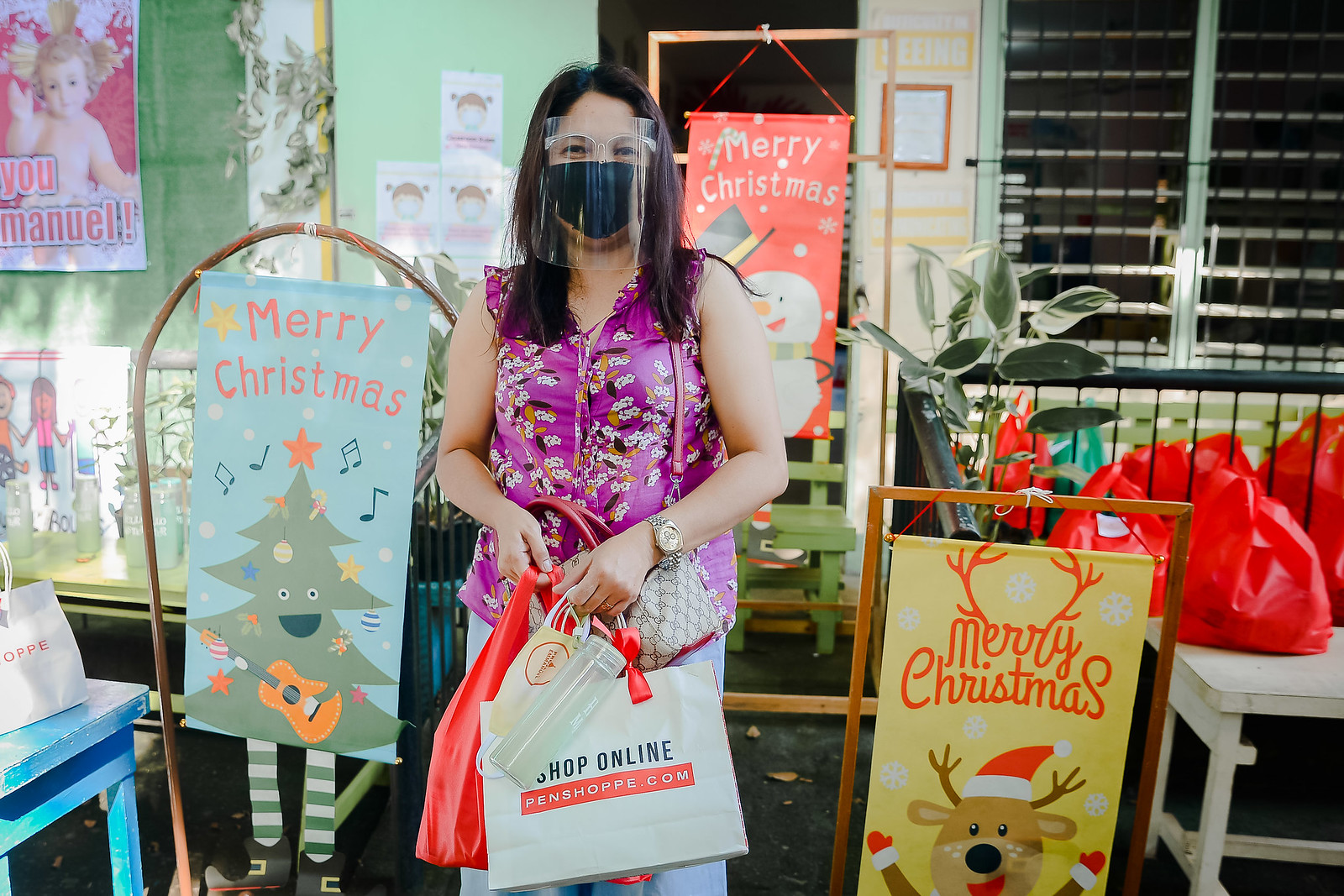A woman with dark brown hair stands on a sidewalk outside a store, wearing a black face mask and a clear plastic face shield. She has on glasses and is dressed in a sleeveless blouse with a purple top adorned with a floral pattern, paired with light blue jeans. In her hands, she holds several shopping bags, including a red one, a white one that says "shop online," and a smaller item that appears to be a bag or a water bottle. Flanking her on both sides are festive stands or banners celebrating the Christmas season. To her left, a banner features a singing Christmas tree with a guitar and music notes, complete with eyes and a mouth. To her right, another banner displays a cheerful cartoon reindeer with outstretched arms, eyes, a nose, and a mouth open in a smile. The overall setting includes multiple holiday-themed images and a window frame in the upper right quadrant, indicating that the scene likely takes place indoors.